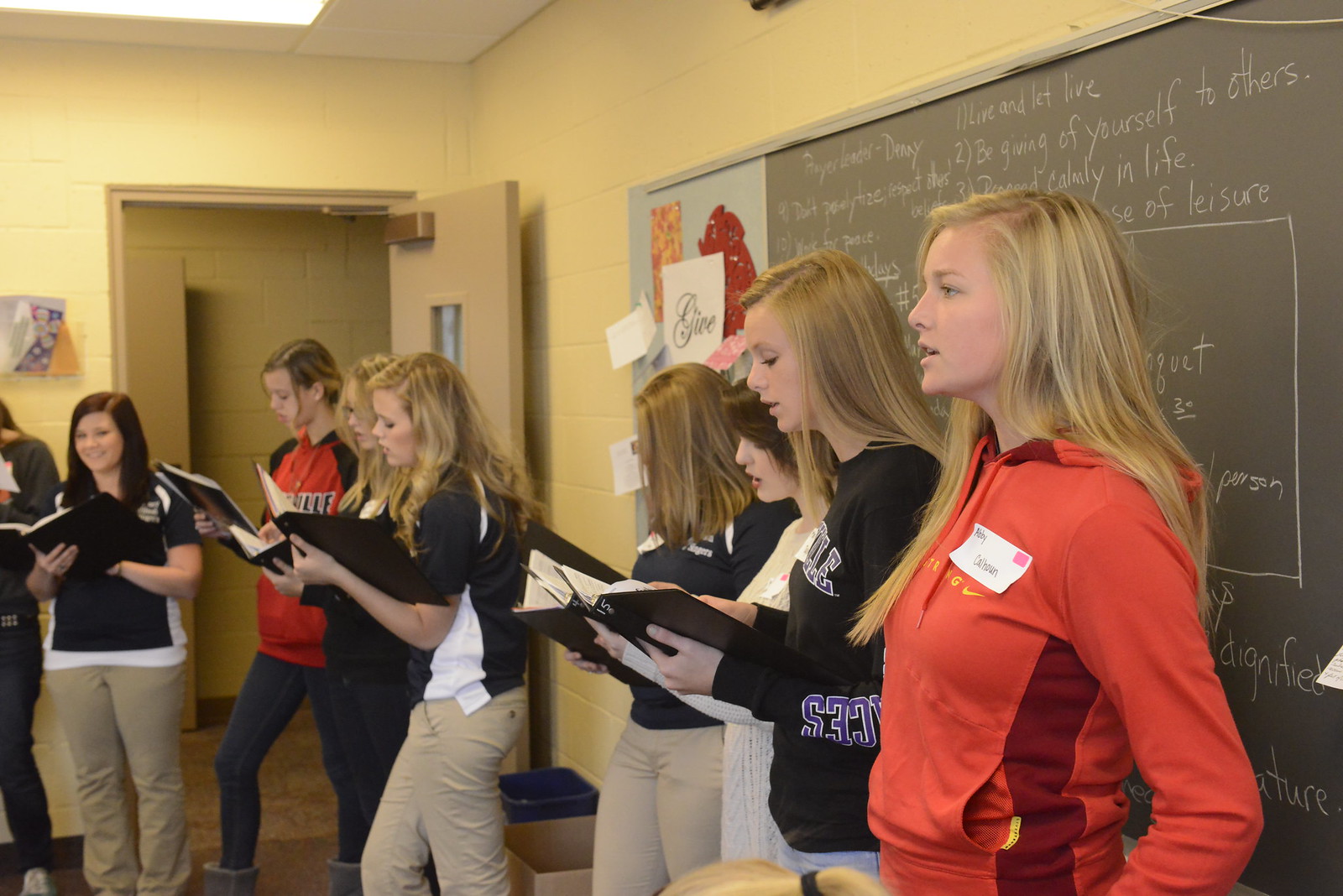In this color landscape photograph, nine high school or college students, predominantly young women with an assortment of long blonde and brown hair, are gathered in a classroom setting. They stand in front of a chalkboard that features extensive white chalk writing and colored illustrations on the left side. Most of them are holding open black binders, from which they appear to be reading or possibly reciting together, while looking towards something or someone off to the left of the frame. The students are casually dressed in various clothing, including T-shirts, khakis, black hoodies, and an array of other sweatshirts and pants. The most prominent figure, positioned to the right front of the image, has long blonde hair and is wearing a red hoodie, distinct from the others as she is not holding a binder and is gazing straight ahead. An open door is visible at the back left of the classroom, adding depth to the scene. The image captures a realistic, representative moment of classroom activity, emphasizing the students' engagement with their binders.